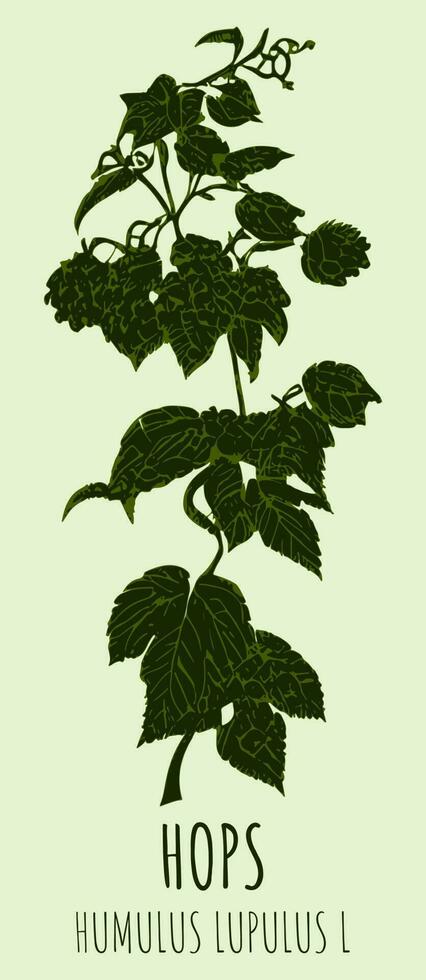The image is a vertically rectangular, two-color print piece depicting hops. The background is a very light mint green, providing a gentle contrast to the darker green elements. At the bottom of the image, the word "HOPS" is prominently displayed in bold, all-capital letters. Directly beneath it, the Latin scientific name "HUMULUS LUPULUS L." is written, also in all capitals but not bolded. Central to the image is an illustration of a green, leafy, vine-like hops plant. The leaves exhibit a rich, ivy-like appearance and cluster more densely towards the bottom, gradually becoming smaller as they extend upwards. The image has no specific border, allowing the artwork to blend seamlessly into the light green background. The overall design is clean and focused, emphasizing the botanical details and the minimalistic text layout.